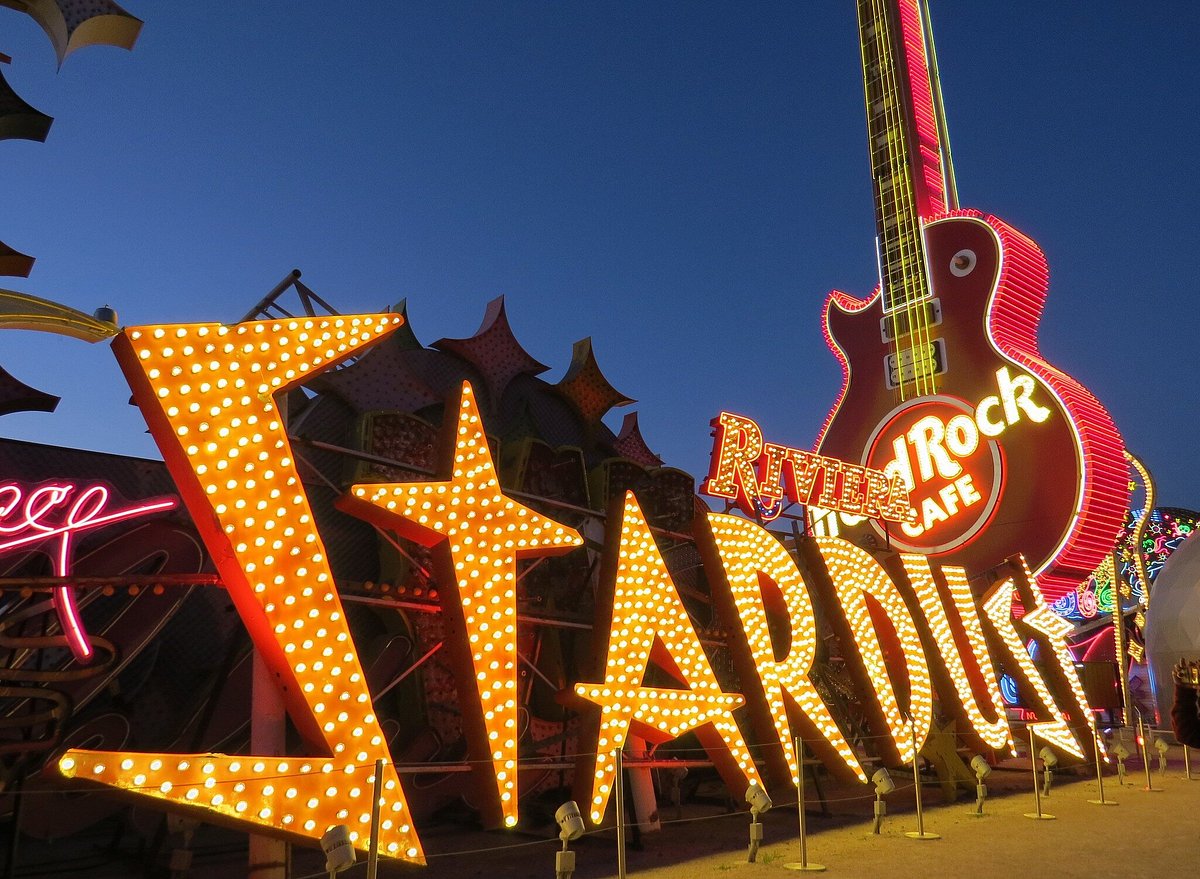This outdoor photograph captures a vibrant scene in Las Vegas, Nevada, featuring iconic vintage casino and restaurant signage under a clear, blue sky. Dominating the image is a massive, red guitar points up to the sky with yellow strings, identified as the Hard Rock Cafe's signature emblem. The guitar is adorned with red LED lights around its walnut-colored body, and its white lettering. In the foreground, a bold and nostalgic Stardust sign stands out, constructed from an array of vintage light bulbs, each meticulously placed in metal frames for every letter. The Stardust sign also includes the word "Riviera," hinting at its historic connection to the famed casino. This eclectic mix of signage is complemented by oriental-style structures in the background, adding to the rich and colorful tapestry of Las Vegas's storied past. The likely setting for these signs is either an exhibit celebrating the history of these landmark establishments or a junkyard dedicated to preserving these dazzling relics.